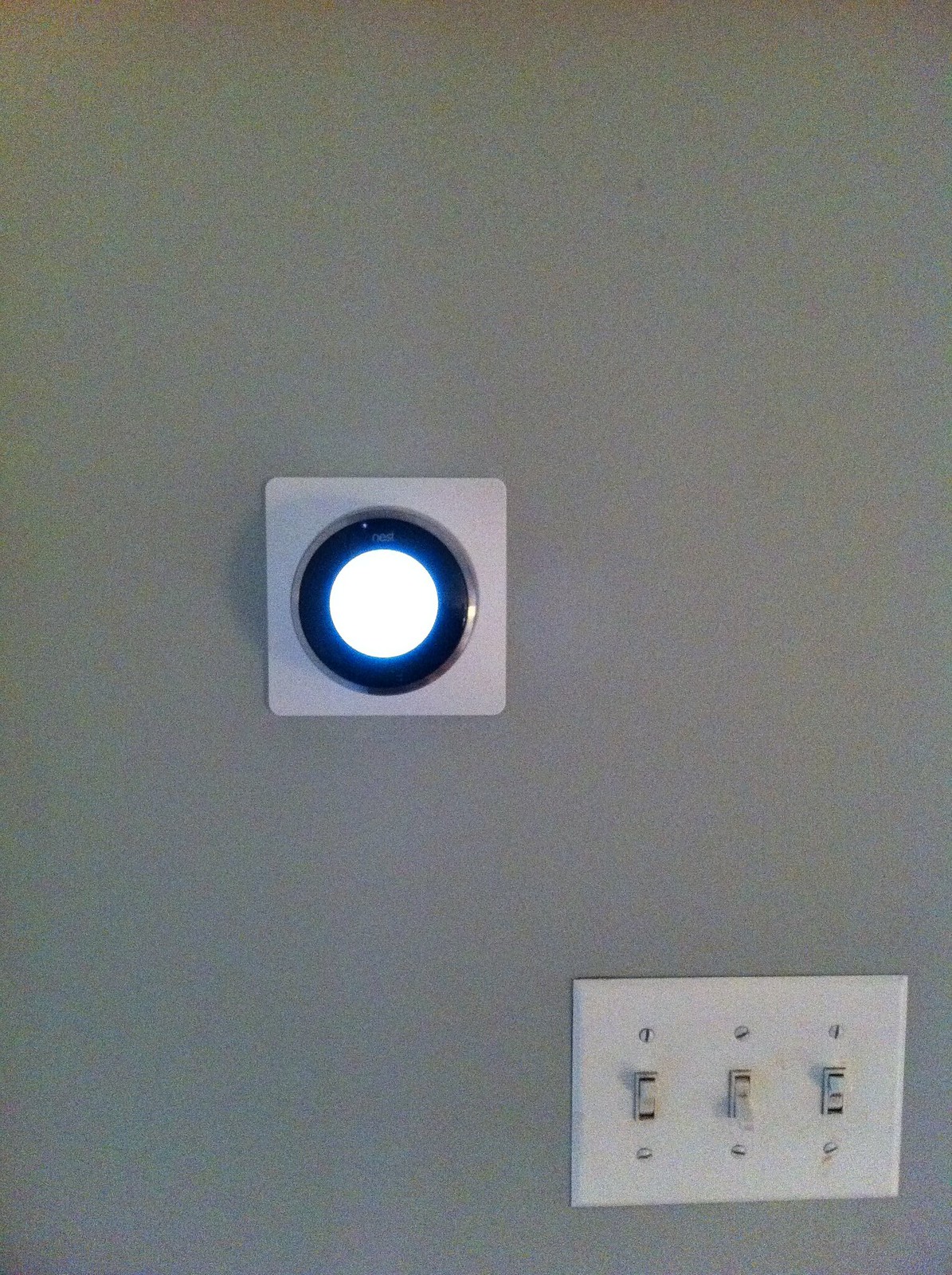The image features a minimalist interior scene focused on a smart home device affixed to a grayish-colored wall, which spans the entire background. Positioned toward the middle-left of the frame is the device, identified as a Nest smart thermostat. This device has a sleek, modern design, characterized by a white square backdrop upon which it is mounted.

The Nest thermostat itself is composed of a circular interface with a prominent silver border. Within this border, a thicker black ring adds contrast and houses the branding; the word "Nest" is clearly displayed in white text at the center. The black ring encircles a very bright white light, possibly indicating that the device is active or in use.

On the bottom-right of the image is a rectangular light switch panel, set against the same gray wall background. This panel contains three individual switches, each with a white base. The switch on the far left is toggled upwards, the middle switch is in the down position, and the right switch is also toggled upwards. Each switch is flanked by white screws positioned at the top and bottom edges of the panel, securing it to the wall.

The composition of the image highlights the integration of smart home technology within a simple, contemporary interior setting.